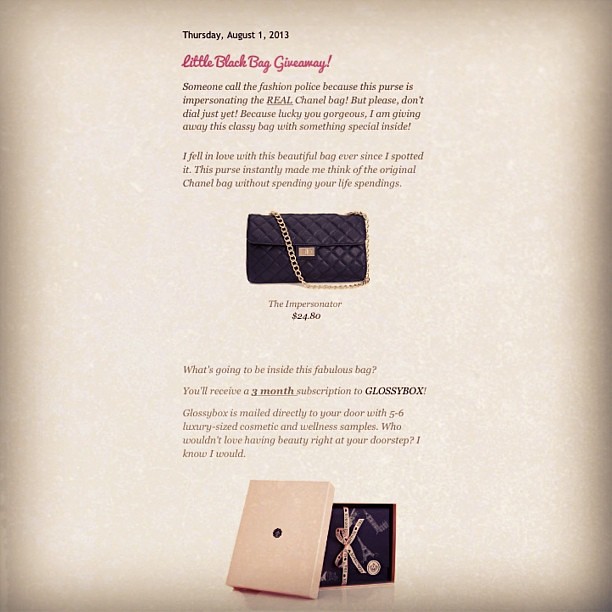This image is an official advertisement with a light brown beige background, featuring a detailed giveaway announcement. At the top in black letters, it reads, “Thursday, August 1st, 2013.” Below that, in red cursive, it says, “Little Black Bag Giveaway.” The central portion of the ad carries black text stating, “Someone call the fashion police because this purse is impersonating the real Chanel bag, but please don't dial just yet, because lucky you gorgeous, I am giving away this classy bag with something special inside.” There’s then a paragraph where the seller expresses their infatuation with the bag, linking its elegance to that of an original Chanel bag, without the exorbitant price. The advertisement presents a black purse with a silver chain handle labeled as "The Impersonator" priced at $24.80. It then excites the reader with further details: inside this stylish bag, there is a surprise gift—a three-month subscription to Glossy Box. Glossy Box delivers five to six luxury-sized cosmetic and wellness samples directly to your doorstep. Who wouldn't want beauty at their doorstep? The ad's color scheme includes black, white, red, and navy blue, making it visually appealing. At the bottom of the flyer, there’s an image of a gift box, accentuating the excitement of the giveaway.